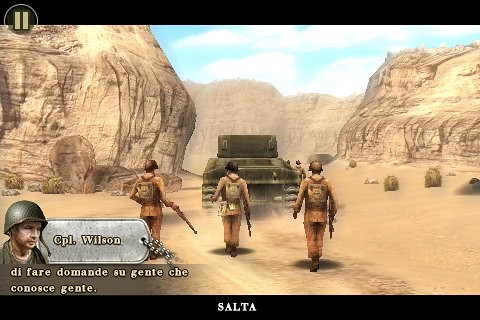In this color screenshot from a video game, the scene unfolds in a desert-like ravine flanked by massive boulder rocks on either side. At the top left corner of the screen, a pause button indicates the game is paused. The game interface features a black bar at the top and bottom, with the bottom bar displaying the word "SALTA" in white text. On the left side of the screen, there's an icon of an army man identified as Corporal Wilson, with dog tags beside him. Below his image, there is text in a foreign language, possibly French, with phrases like "die fair," "mon su junta," "a chief con," and "say gente." The gameplay itself shows three soldiers dressed in camo uniforms and helmets, each carrying weapons and wearing backpacks, walking behind a tank. They're navigating through the dusty ravine under a bright blue sky dotted with fluffy clouds. The surreal yet detailed animation vividly captures the rugged terrain and military-themed atmosphere.